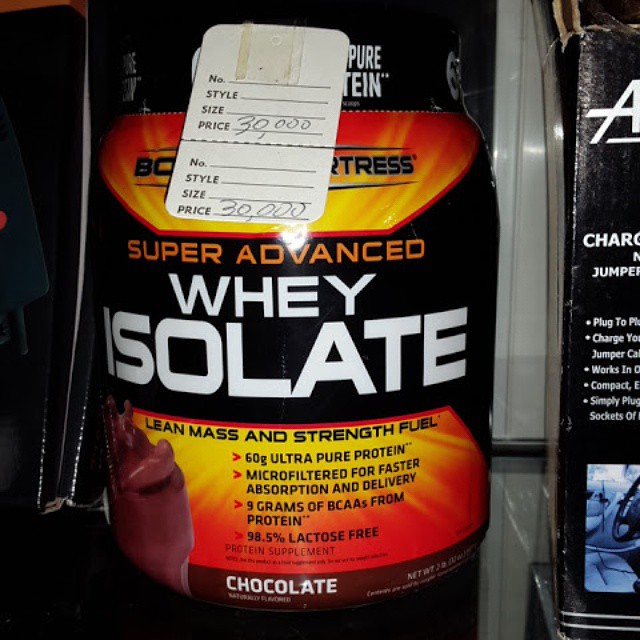This image showcases a container of protein powder, specifically the "Body Fortress Super Advanced Whey Isolate." The container features a prominent red and black design with a hint of yellow. The label details various product attributes, including "60 grams Ultra Pure Protein, Microfiltered for Faster Absorption and Delivery," "9 grams of BCAAs from Protein," and "98.5% Lactose Free." Additionally, it states "Lean Mass and Strength Fuel" in black text. The flavor is indicated as chocolate, presented in a black rectangle at the bottom. Adjacent to this, there's an illustration of a brown chocolate shape. The price is marked at $30,000, though the currency is unspecified. The setting appears to be an indoor shop, with various items and accessories in the background.